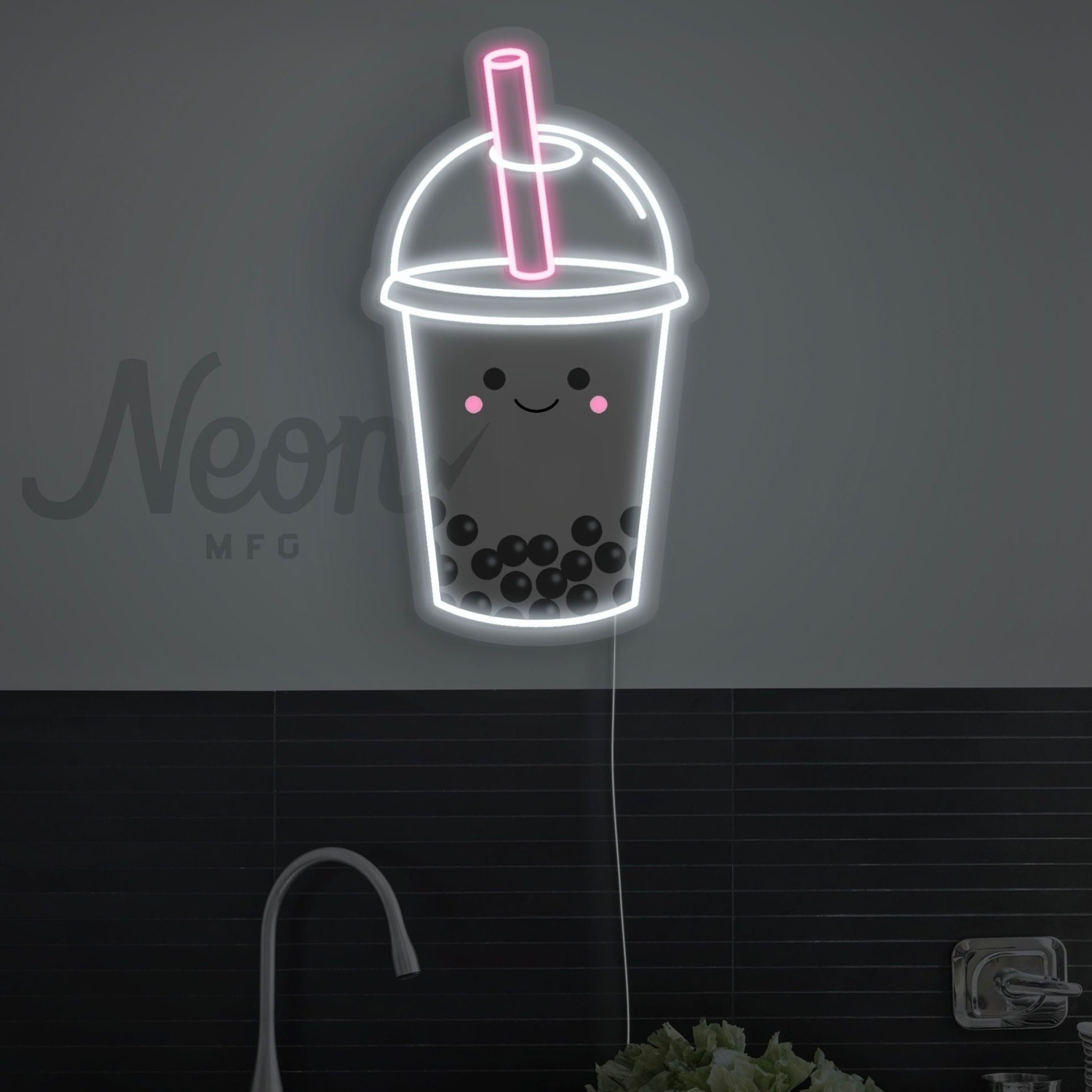This is a digital illustration depicting a dimly lit, square-shaped scene inside what appears to be a restaurant or café. The central focus of the image is a glowing neon light sculpture in the top center, shaped like a happy cup of boba tea. The cup is outlined in white, with black boba balls at the bottom, a neon pink straw extending from the top, and a smiley face complete with pink dimples. The word "neon MFG" is written in a fancy cursive neon style on the left side of the image, slightly darker gray against a flat gray wall. This gray wall occupies the top two-thirds of the background, while the bottom third is composed of black-painted bricks. Near the lower part of the image, there is a dark partition where a sink spout and a plant—possibly lettuce or kale—are barely visible. The overall dark tones of the image accentuate the bright, eye-catching neon cup, making it the most prominent feature in this visually intriguing scene.